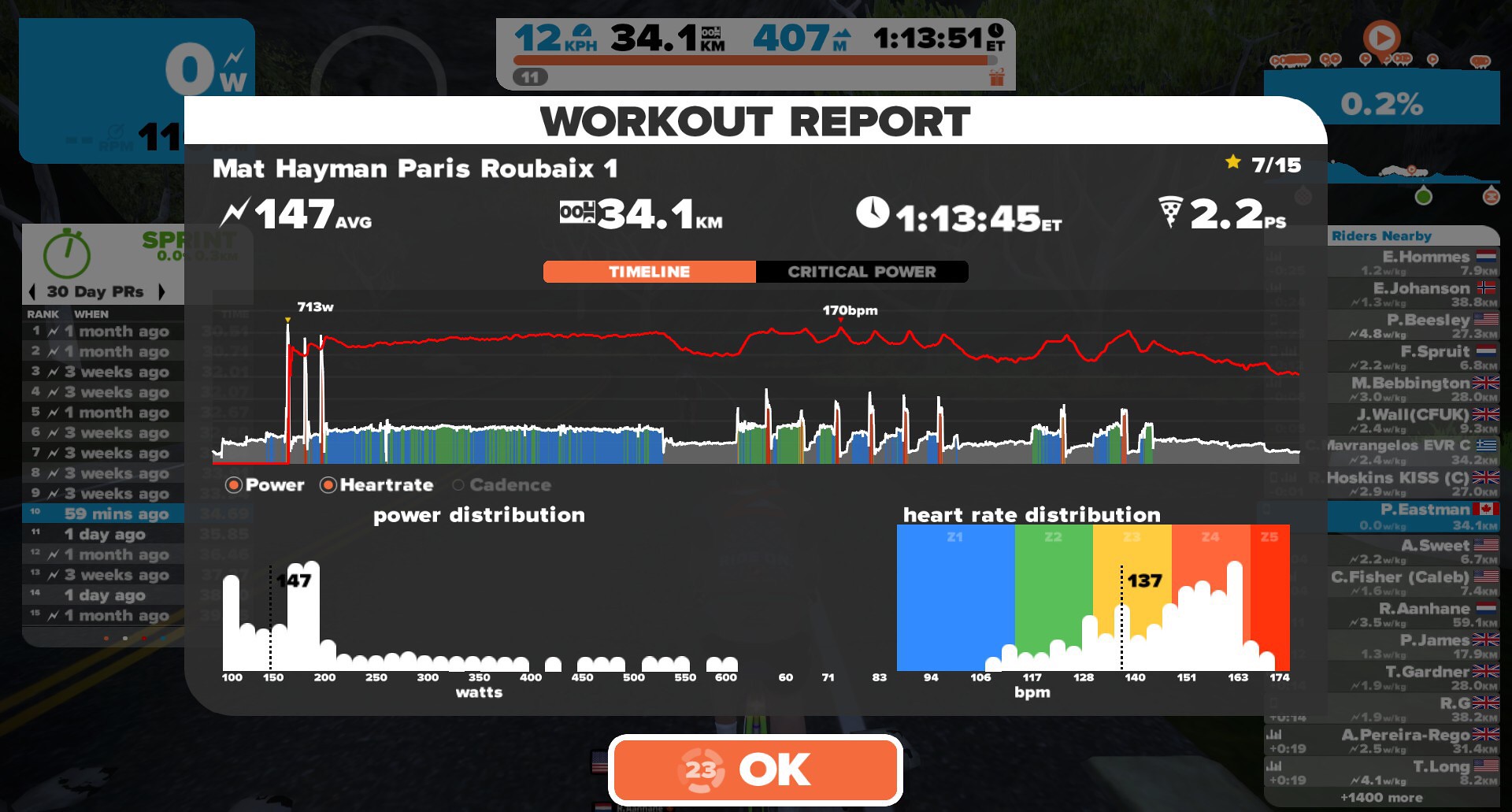The image is a detailed screenshot of a workout application's interface, prominently featuring a 'Workout Report' window. The report window is titled with "Workout Report" in bold black text on a white banner at the top. Below this, the user's name, Matt Heyman, is displayed alongside location details, "Paris, Round the Knicks." The interface is rich with statistical data including heart rate, distance, time, and specific numeric values such as 147, 34.1, 113, 45, and 2.2.

The main content consists of multiple charts and graphs. In the center, there's a color line art graph with metered readings and a red response line. On the bottom left is a white column or table labeled "Power Distribution," and to the bottom right is a colorful chart marked "Heart Rate Distribution.” The charts use a variety of colors including black, red, blue, green, yellow, and orange, organized in a symmetrical layout. Text and numbers align primarily from left to right, culminating in an orange horizontal bar at the bottom center with white text reading "Okay." The overall style of the image is a color illustration infographic, blending clear numerical data with vivid graphical elements.